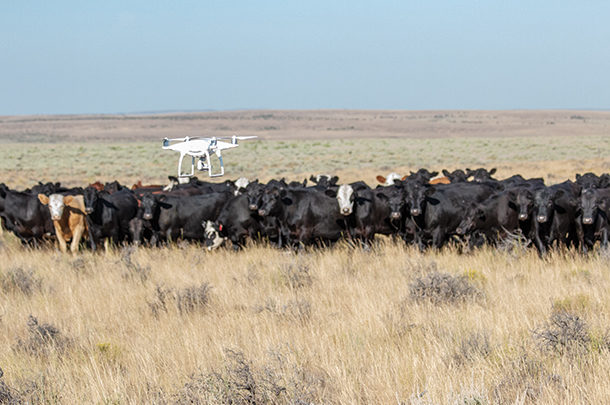In this image, a large group of cows, predominantly black with a few white-faced and light brown individuals, occupies a vast open field. The field features a variety of terrains, transitioning from tall, straw-like, light brown grass in the foreground to mixed patches of lighter green and brown vegetation. The backdrop includes a blue horizon that gradually melds into a grayish sky without any visible clouds, and faintly discernible low mountains. A white drone with four propellers hovers to the left, seemingly used to herd the cows. These cows form a dense, centralized cluster extending horizontally across the image, suggesting a sense of motion and organization within the open expanse.